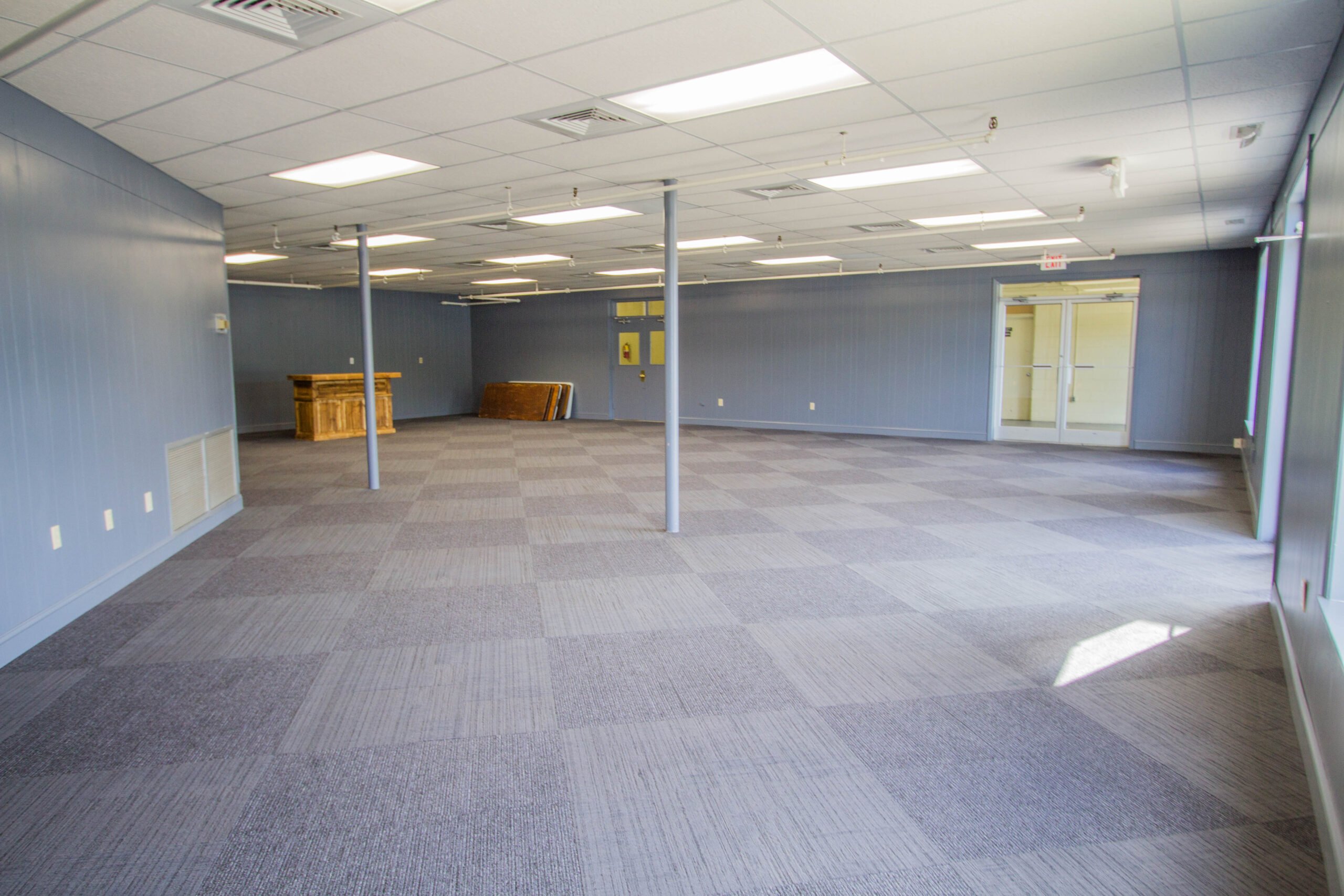The image depicts an empty commercial space, likely an office or foyer, characterized by a checker-patterned carpet composed of alternating dark gray and lighter gray squares. The walls are painted a lighter blue, aligning with the hues of the carpet, creating a cohesive color scheme. White panel ceilings with rectangular fluorescent lights give a traditional office ambiance, and the ceiling appears relatively low. The room features several posts extending from the floor to the ceiling. On the left side, there are clear double doors marked with an exit sign, along with a couple of wooden furniture pieces and smaller windows. The right side includes another window, allowing a trickle of sunlight to filter through. Toward the back, there is a wooden bar or podium, standing alone against the wall. The overall setting suggests a recently vacated space, awaiting new occupants.